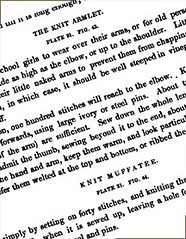The image is a small, blurry screenshot of a printed page, which appears to be part of a detailed description of knitting wear, specifically for schoolgirls. The text is at an angle, rising from left to right at about 10-15 degrees. The first paragraph describes the "knit armlet," designed to be worn from the elbow up to the shoulder to keep the arms warm and prevent chapping, potentially treated with vinegar for added protection. It mentions using ivory or steel pins for knitting 100 stitches to reach the elbow, incorporating a thumb hole for a snug fit around the hand and arm. The armlets are noted to be welted at the top and bottom or ribbed. The second paragraph is partially visible and titled "knit muffety," but the text is cut off on both sides, making it difficult to read. The page is printed in black text on white paper, structured into several photographic plates with descriptive paragraphs.